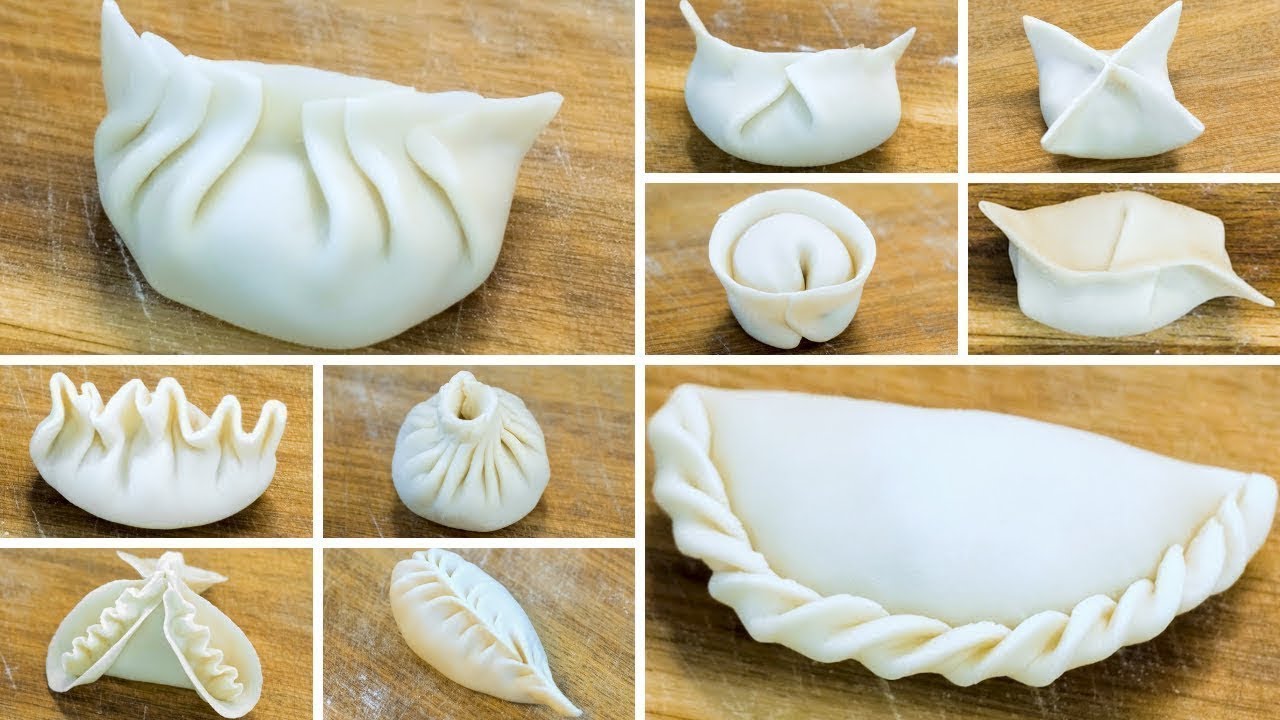The image displays a comprehensive collage featuring variations in dumpling and wonton folding patterns. The collage is organized into ten distinct photographs, arranged in a grid format. Situated prominently, two large images occupy the top left and bottom right corners, exhibiting intricately designed dumplings or wontons of similar size and detail.

Below the large image on the left, four smaller pictures are elegantly laid out in two rows and two columns, each showcasing unique folding techniques and patterns. On the right side, surrounding the large image, there are also four smaller images positioned in a similar 2x2 grid, revealing additional folding styles.

The dumplings and wontons depicted appear traditional, with some featuring perforations as part of their design. The collage does not include any skewers or sticks, emphasizing the classic, hand-folded appearance of each dumpling or wonton. The visual presentation offers an informative array of artistic and culinary craftsmanship involved in preparing these timeless delicacies.